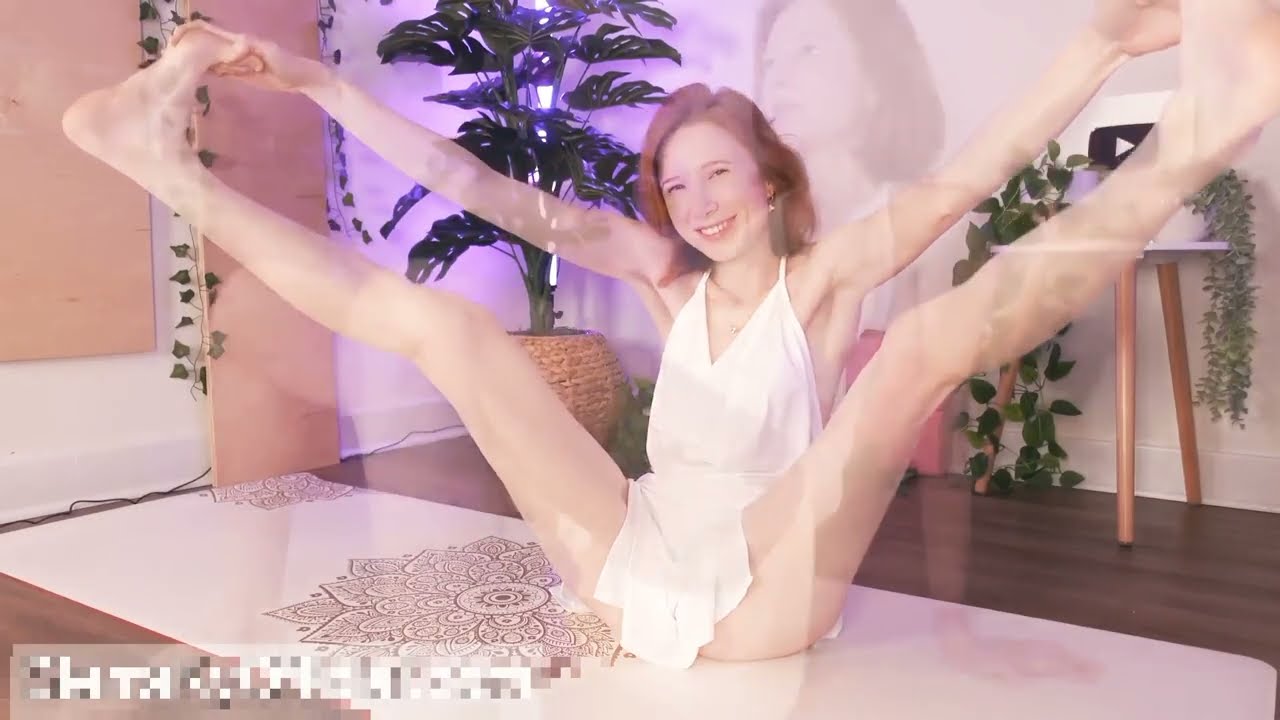In a serene yoga studio with a light beige interior and a hardwood floor, a tall, pale-skinned woman with reddish-brown hair is captured in a complex pose. She is sitting on a white yoga mat that features a brown floral design, dressed in a tight white outfit, possibly a dress or bathing suit, which covers her private areas but reveals much of her form. With her legs extended upwards in a wide V-shape, she holds her feet with her hands and smiles gently at the camera. Behind her, an array of greenery creates a tranquil vibe, including a large plant in a tan wicker basket positioned in the left-hand corner and another plant draping gracefully from a white table with tan legs on the right. A ghostly second image of the woman appears faintly in the background, adding a mystical element to the scene.